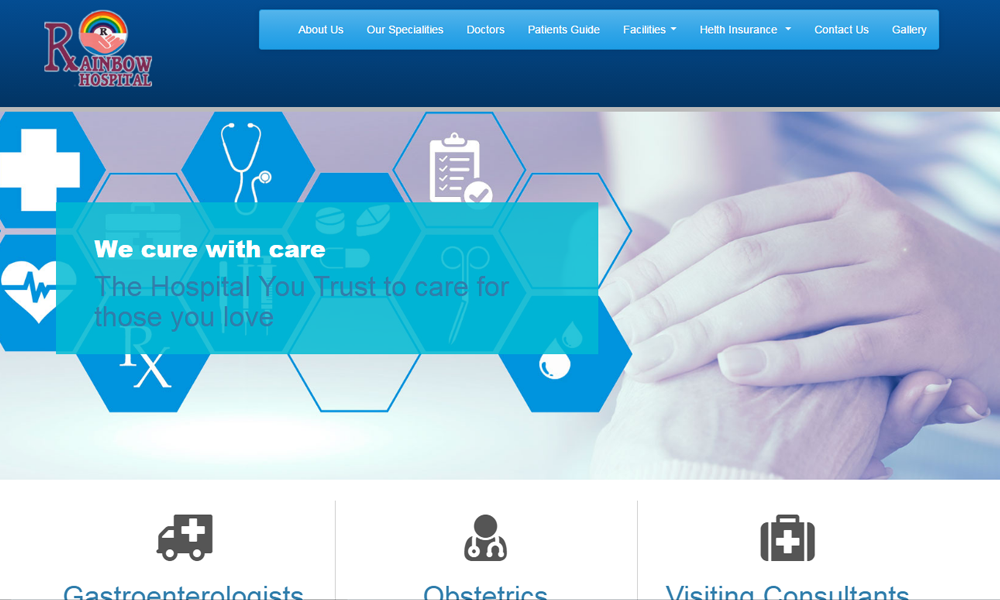Here is a cleaned-up and detailed descriptive caption:

---

The image appears to be a screenshot of a hospital's website, specifically "Rainbow Hospital." 

**Top Section:**
- In the top left corner, "Rainbow Hospital" is prominently displayed with an exceptionally large 'R'.
- Adjacent to the large 'R' is an icon within a circle, representing a rainbow with the bottom arc forming the shape of a hand.
- This text and icon sit on a solid dark blue background that spans horizontally across the entire width of the image.

**Navigation Bar:**
- Towards the right side of this dark blue horizontal background, there is a light blue rectangular section containing white text. From left to right, the text includes:
  - "About Us"
  - "Our Specialties"
  - "Doctors"
  - Two indistinct sections with text that is illegible due to its small size, one of which has a dropdown arrow.
  - "Facilities" with a dropdown arrow
  - Another illegible section with a dropdown arrow
  - "Contact Us"
  - "Gallery"

**Main Banner:**
- Beneath the navigation bar is the main banner of the website.
- On the right side of the banner are two clasped hands symbolizing care.
- To the left side, horizontally stacked hexagons resembling a beehive pattern are displayed. These hexagons feature varied backgrounds—some transparent and others shaded dark or light blue—and contain white icons representing healthcare-related items such as an 'RX', a checklist, and a stethoscope.

**Icon Section:**
- Below this, there are three icons evenly spaced:
  - On the left, a gray and white ambulance
  - In the middle, a doctor with a stethoscope draped over their shoulders
  - On the right, a first aid kit
- Blue text is positioned underneath these icons, though the text is partially cut off and not fully readable.

This comprehensive layout reflects the key visual elements and primary navigation options of the "Rainbow Hospital" website, combining healthcare imagery with user-friendly navigation features.